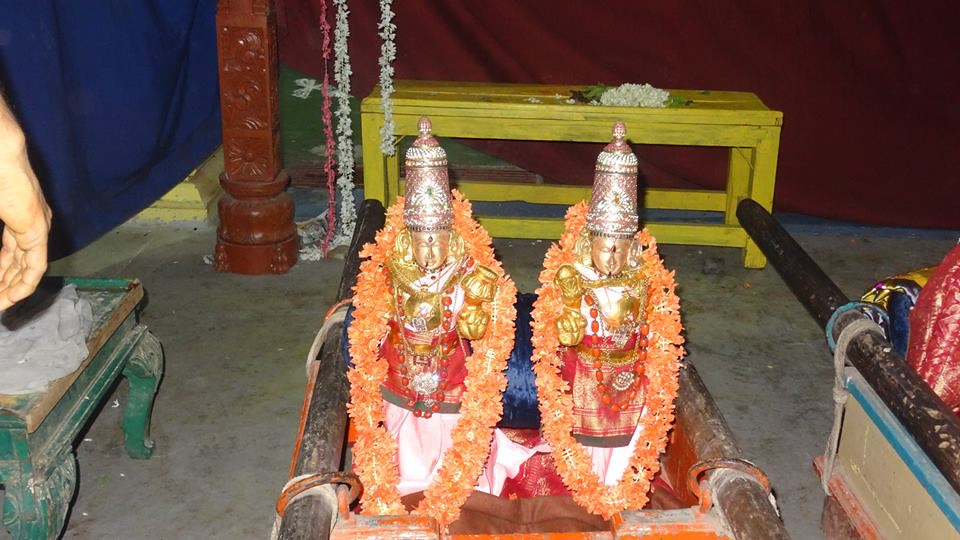The image captures an indoor scene resembling an old-school temple with a cement floor. On the left side, a blue curtain hangs, while a prominent red curtain dominates the middle. In front of this red curtain stands a yellow table adorned with white flowers. Positioned before the table are two elaborate statues, which appear to be golden and possibly represent Hindu gods or revered figures like Buddha or the Dalai Lama. Each statue is crowned, clothed in intricate red and gold garments, and encircled by an orange wreath of flowers. The statues exhibit detailed craftsmanship, with gold skin and adorned with beads and intricate gold patterns. Surrounding the statues are additional elements like a chair on the left and a yellow bench.